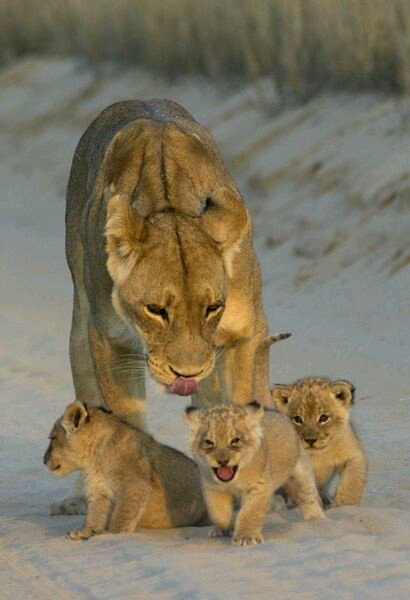In this detailed photograph of wildlife, we see a female mountain lion, distinguished by her golden-brown fur and a striking black stripe that runs from between her eyes down her neck. She stands protectively behind her three fuzzy cubs in a snowy landscape. The snow covers the ground and a small hill in the background, giving a serene wintry setting. The mother lioness has her tongue licked out, possibly licking her lips. Of the three cubs, one is sitting to the left, looking away from the others, while the middle one is standing with its mouth open, almost appearing to smile. The third cub on the right sits calmly, looking straight ahead. Each cub shares the same golden-brown hue as their mother, blending harmoniously with her in this beautifully captured moment of nature.